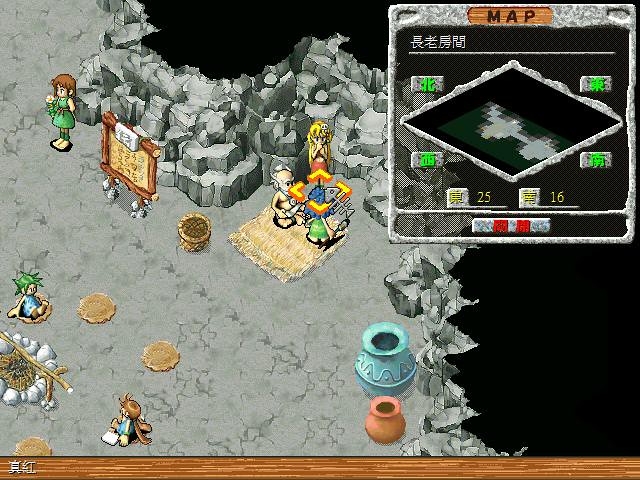This screenshot from a video game features a detailed scene set in what appears to be a cave, indicated by walls lined with dark and light gray rocks. Central to the display is a diamond-shaped map located in the upper right corner, showcasing unexplored areas in black and explored paths in gray and white squares. The map includes four gray rectangles with Japanese writing in lime green at each corner and additional numeric and Japanese text at the bottom, highlighted in yellow. Within the screenshot, multiple anime-style characters are dispersed. There's a notable group seated on a wicker rug: an old, shirtless man with gray hair holding an object, a person with blue hair featuring floating fish bones, and a green-haired individual in a blue dress. Near a fire pit with gray stones and black coals, a cylindrical piece of wood, and many unlit sticks, sits another set of characters: a green-haired girl in a blue shirt and a brown-haired girl in a blue dress. Standing nearby, a short-haired girl in a green dress adorned with a red rope around her waist holds a white flower with an orange center. The characters are surrounded by various items, such as a tan sign bordered with brown wood featuring Japanese text and a wicker basket with round contents. The image also displays numerous colorful vases, including a cyan blue vase and a brown one with a red top. The area is well-detailed, right down to the light and medium brown wooden flooring, with an additional gray area and spots of tan lining the edges, contributing to the intricate, immersive environment depicted.